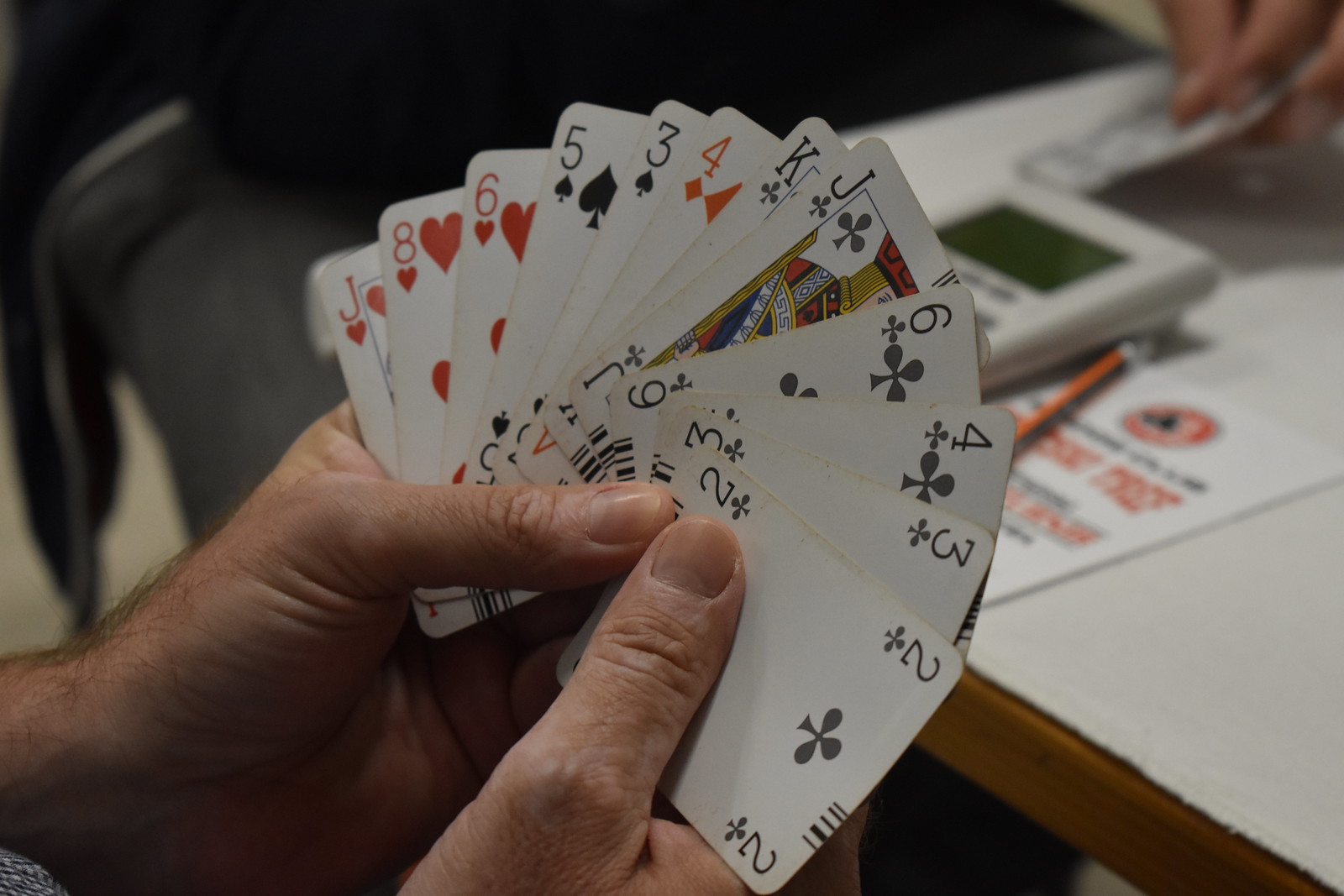In the image, a person is holding a hand of playing cards, both hands fanned out with thumbs touching. The cards in hand include a Two, Three, Four, Six, Jack, King of Clubs, Four of Diamonds, Three and Five of Spades, and Six, Eight, and Jack of Hearts, suggesting a game where order and suit matter, such as Hearts or Rummy. The cards appear well-worn, implying frequent use. Behind the cards, the front of the person's hands is visible, obscuring the back. 

The setting includes a white tabletop, likely a counter, with a calculator or similar device in the background. A blurry figure across the table appears to be laying down a card or a small stack of five or six cards. In front of this person is a piece of paper with a red logo and red writing, and a standard yellow number two pencil lying across it, indicating a serious game with score-keeping. The table itself is made of yellow pine wood beneath the white top.